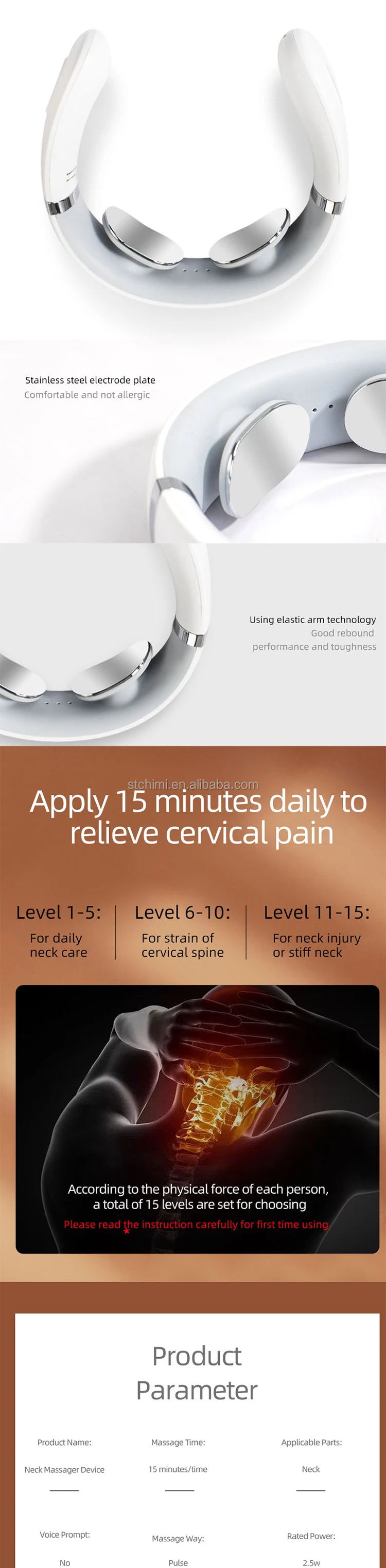This image captures a mobile device displaying a website, specifically stchimi.en.alibaba.com, which appears to be a condensed version of a full webpage, resulting in some text being difficult to read. The focal point of the website is a white wearable device, presumably for the neck, head, or arm, featuring two massage nodes at its center. Beneath the image of the device, there is a bronze-colored informational box detailing its use: "Apply 15 minutes daily to relieve cervical pain." The description further specifies that the device offers 15 adjustable levels tailored to the user's physical force. A red notice advises first-time users to carefully read the instructions. Additionally, there is an illustrative image highlighting the neck area with an overlaid hotspot indicating pain relief. At the bottom of the screen, a white box labeled "Product Parameter" provides detailed specifications of the device.